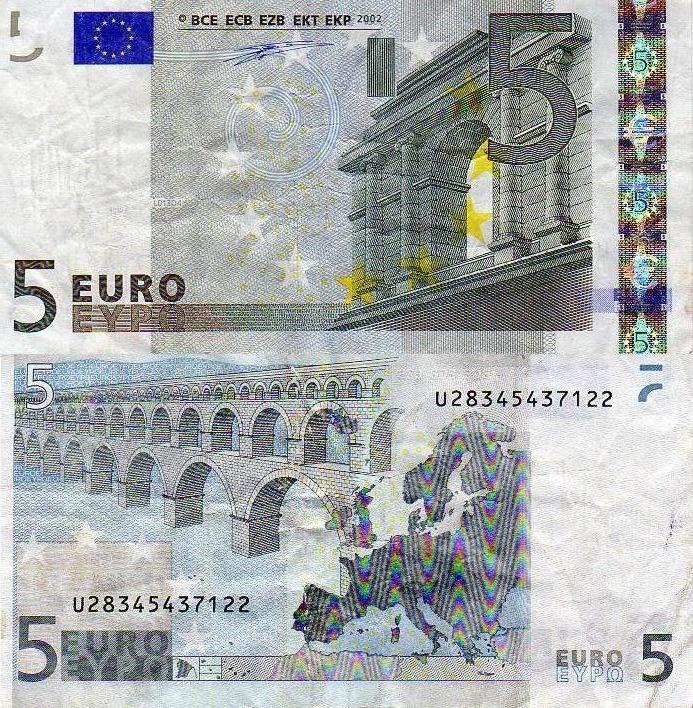This close-up image features both the front and back of a 5 euro bill from 2002. The front side is dominated by a detailed illustration of a stone window, symbolizing classical European architecture. In the top left corner, there's the blue flag of the European Union with a circle of white stars. Each corner of the bill is marked with the number '5'. Alongside the portrait, there's an intricate security strip running vertically, shifting in colors from blues and yellows to reds and greens. The text "Euro-Upo” is visible at the bottom, flanked by the bill's serial number, U28345437122, which repeats at various points. 

On the back, the number '5' is also present in each corner and the bill's serial number appears both at the bottom left and top middle. The central image is a stylized depiction of a bridge, which symbolizes a channel bridge connecting different parts of Europe. The background features a map of Europe, unifying the design elements. The bill maintains a color scheme of grays, blues, and whites, with some yellow stars adding a touch of color. Key elements such as pillars, the EU flag, and text including 'BCE, ECB, EKT, EKP' and the omega symbol add further authenticity and security to the note.